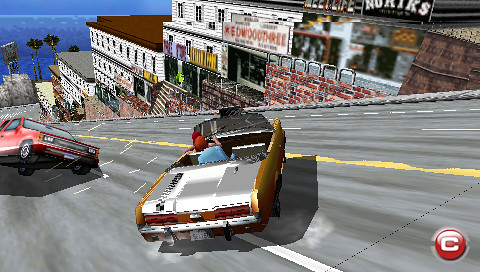In the still image taken from a video game, the scene features a character navigating a gold-colored convertible car with a white trunk down a steep hill. The street, rendered in gray asphalt or concrete, is lined with various buildings, stores, and restaurants, adding to the bustling urban atmosphere. In the background, the serene blue sky and pixelated blue ocean create a striking contrast against the tropical palm trees swaying gently. Adding to the sense of action and tension, an oncoming red car is dramatically pitched on two wheels, suggesting either a crash or a high-speed race. The combination of these elements creates an immersive and dynamic scene within the game.